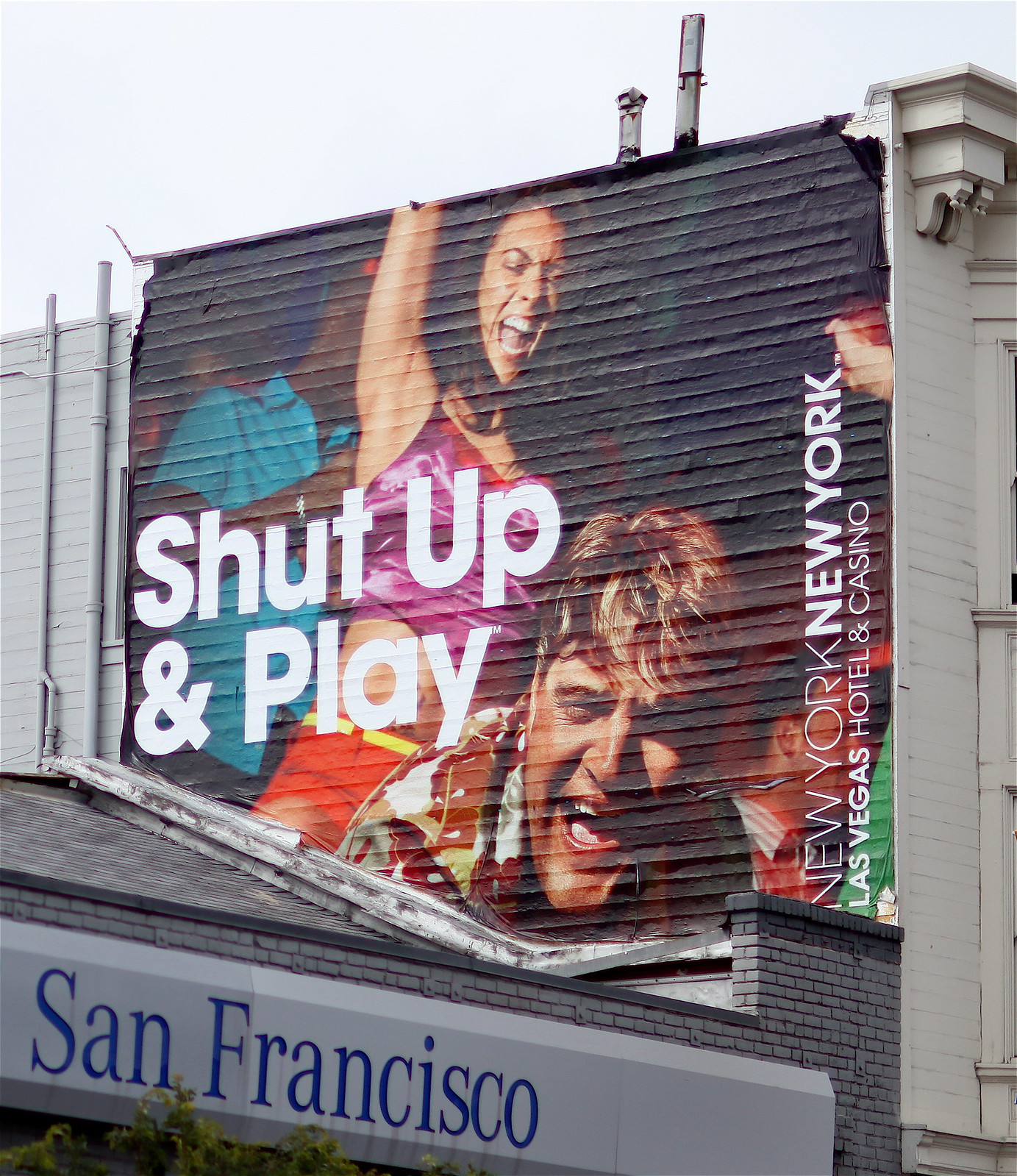The image features a large billboard affixed to the side of a gray brick building in San Francisco, where the advertisement is more like a thin, pasted paper. The bottom of the billboard aligns with the top of the photograph, which shows the upper portion of the building. The building has "San Francisco" written in thin, curvy blue letters across it. 

Visible in the frame is the top of a tree near the building's base and the structure itself is composed of about 30 lines of bricks, indicating its considerable size. Above the building, a few long pipes protrude from its top and side. There is a glimpse of the building's front, showcasing some detailed architectural work.

The prominent billboard features a vibrant and lively scene where a woman appears to be enjoying herself. She's depicted with her mouth open in laughter, arm lifted high, wearing orange shorts with a yellow belt and a small purple top. Positioned closely in front of or atop a man, she adds to the dynamic energy of the image. The man in front has a delighted expression, mouth also open, and dons a floral print shirt. 

Behind the woman is a black man sporting a blue shirt, holding an object that isn't clearly distinguishable. Additionally, other figures are partially visible to the far right of the frame. The main tagline on the billboard reads "Shut Up and Play" in bold white letters. Running vertically on the right side of the billboard are the words "New York, New York Las Vegas Hotel and Casino" in a sideways orientation.